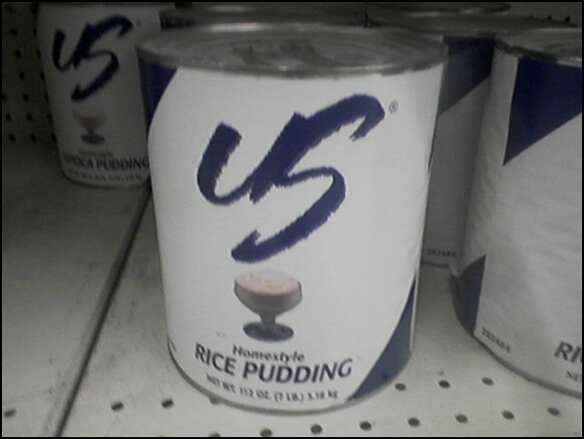The photo captures an up-close, detailed view of a supermarket shelf displaying cans of Homestyle Rice Pudding. On the left side of the image, a can in the distance features a distinctive white and blue design with the prominent letters "U.S." at the top, followed by "Homestyle" in smaller blue lettering, and "Rice Pudding" below it. The can also indicates the net weight as 12 ounces. Below the text, there is an illustration of a small cup filled with pudding. The primary can, positioned centrally and closest to the camera, reveals additional details like its silver top. To the right, two more cans with similar white and blue designs are partially visible, extending off-screen. The shelving itself has perforations, typical of retail store fixtures, with visible rows of holes across its surface. The background wall is white and also perforated, aligning with the store's shelving theme.